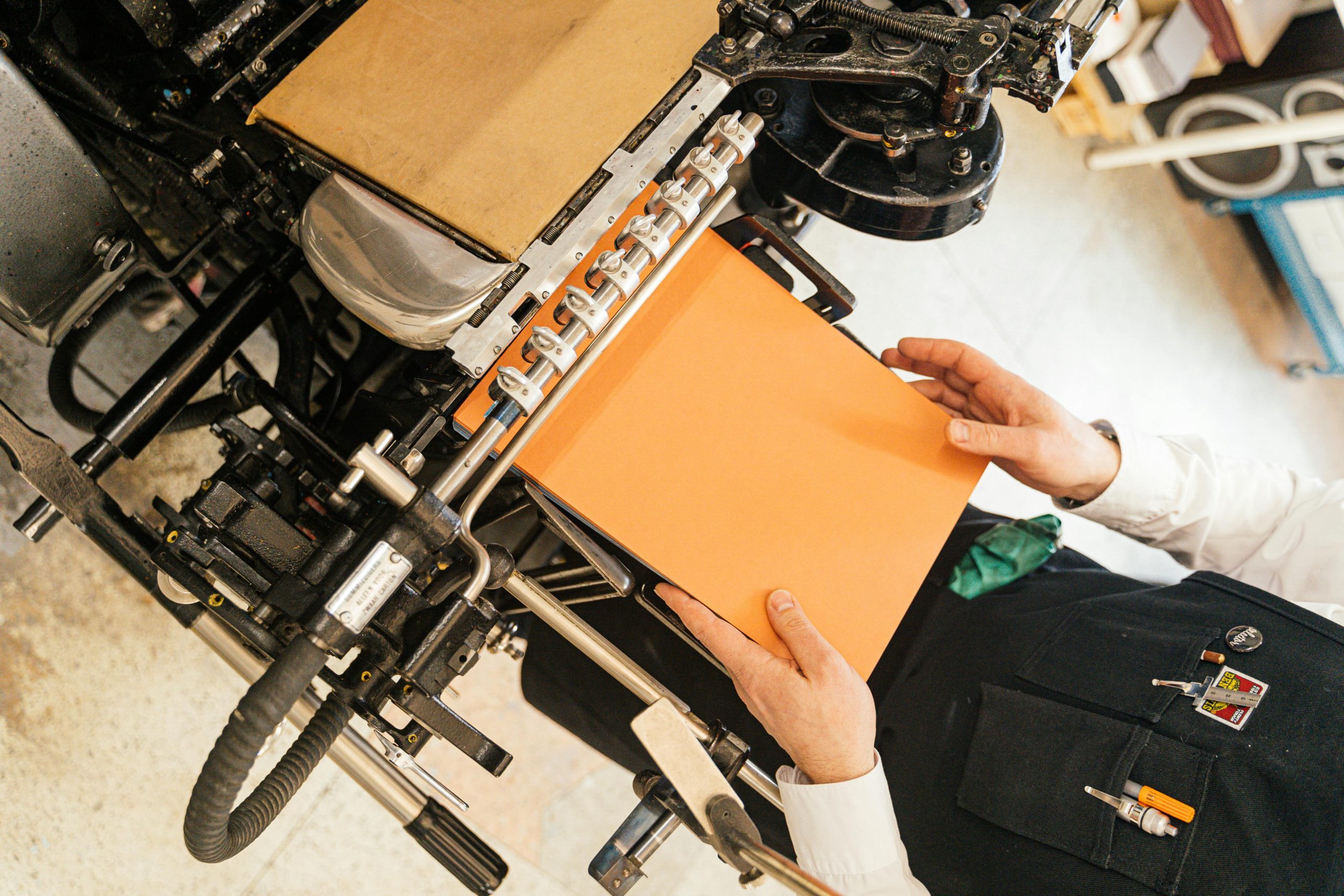The photograph captures an indoor setting, likely a garage, with a man operating a machine, possibly a printing press. The image is rectangular, approximately six inches wide and three inches high, taken from an elevated angle. The man, who appears to be of Caucasian descent, is seen from the chest down, emerging from the lower right corner. He is wearing a black apron with pockets holding pencils, over a long-sleeved white shirt. His hands, bent at the elbows, are outstretched in front of him, handling a stack of papers. The top sheet is orange, with subsequent sheets in gray and blue tones. In front of him sits the machine, flanked by intricate components including a black circular design with gears and a long narrow bar extending towards a black tube or hose on the left. Another bar with a black handle also features on the left side. The floor beneath is a blurred light cement color, and a stereo can be seen in the blurred upper right corner. The color palette includes orange, black, gray, green, red, and blue, adding to the detailed composition of the scene.